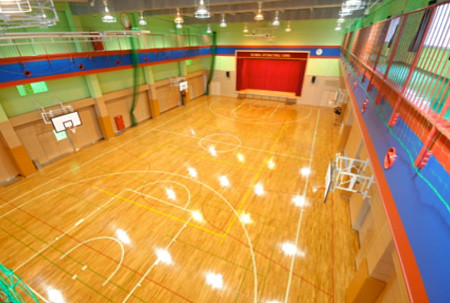This photograph captures the interior of a gymnasium from a vantage point on the second floor, offering a comprehensive view of the space below. The gym's walls are painted in a mint or lime green color, accentuated by a blue and red stripe running around the middle, between the first and second floors. The gymnasium floor is a glossy wooden surface, reflecting the overhead lights beautifully. In the gym, there are four basketball hoops with white backboards positioned on the sides of the basketball court. Down below, a focal point is the stage featuring a red curtain framed by red wooden trim. A metal walkway with an orange gate is visible on the second floor, adding to the gym's structural details. The image provides a well-lit and vibrant view of the gymnasium, highlighting both its practical and aesthetic elements.